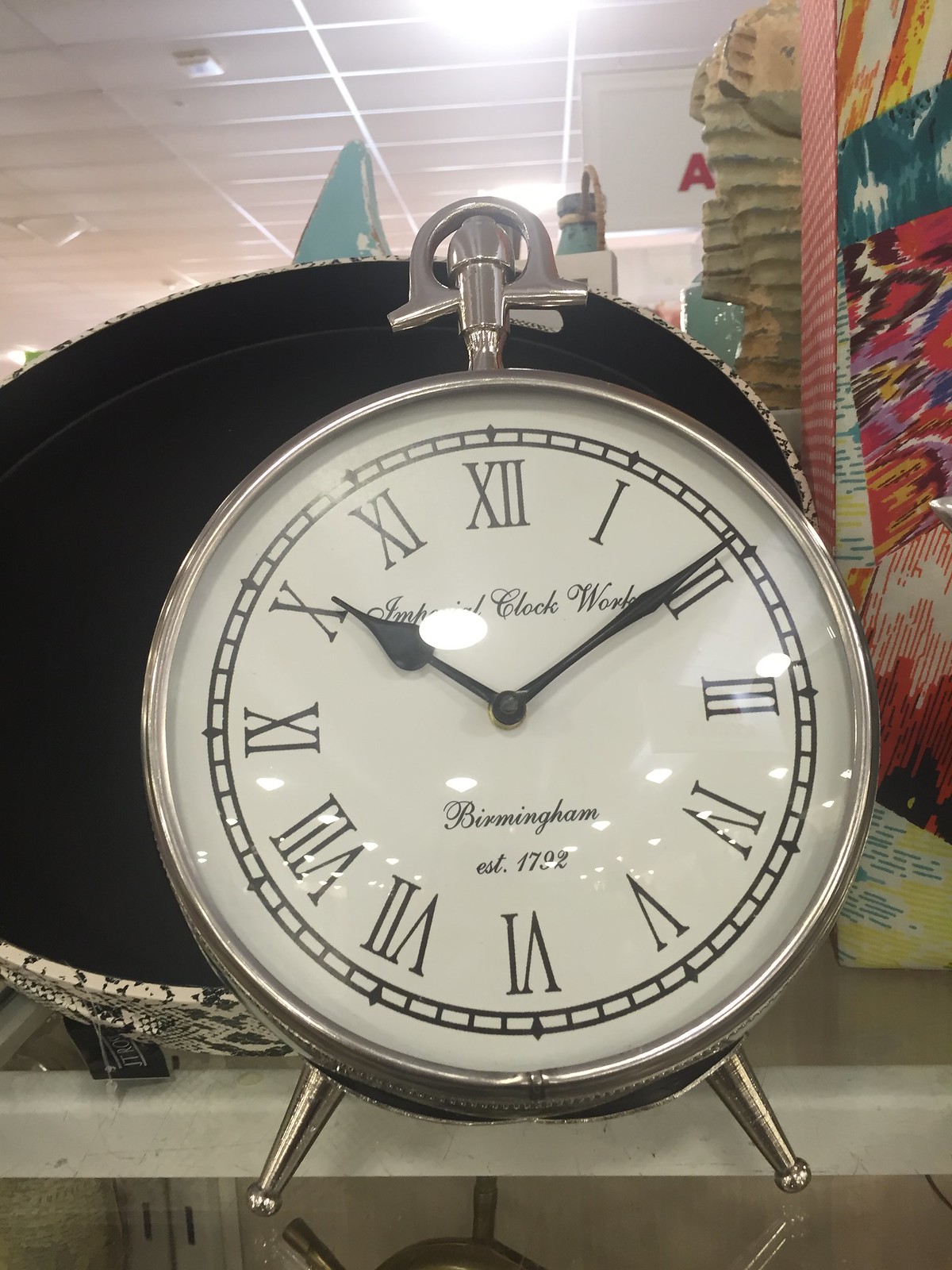This is a photograph of a large, silver, portable clock that resembles a giant pocket watch. Positioned on a glass shelf with white metal supports, the clock features a prominent silver frame and feet. Its design includes a distinctive silver hook-like structure on top, reminiscent of where it would attach to a chain and the knob used to change the hands. The clock face is white, accented with black Roman numerals and bordered by a thick black design. Noteworthy inscriptions include "Imperial Clockworks" in cursive above the center and "Birmingham, established 1792" below it. The short hand points at 10, while the long hand points at 2. The background reveals a mix of colored materials in shades of red, purple, yellow, orange, and black, with the reflection of the clock visible on the glass surface.